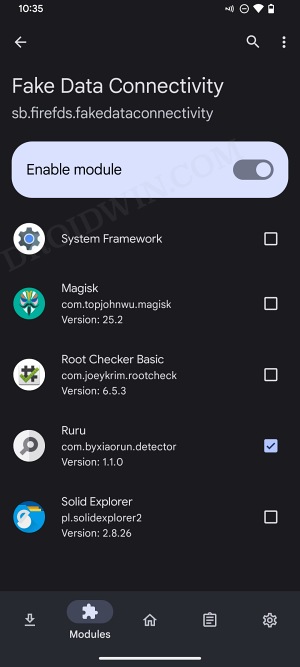The image depicts a settings page on a smartphone. In the upper-left corner, the time is displayed as 10:35. The upper-right corner features the "Do Not Disturb" icon, along with the Wi-Fi and battery icons. Below these indicators, there is an arrow search button. Beneath this button, white text reads "Fake Data Connectivity," followed by a web address: sb.firefds.fakedataconnectivity. 

The central part of the screen showcases a blue box with the label "Enable Module," accompanied by a toggle switch that is currently set to the right, indicating it is enabled. Below this, there is a gear icon next to the text "System Framework," with an unchecked white box to its right. The next item listed is "Magisk," followed by the package name "com.topjohnwu.magisk" and version number "2.5.2," also with an unchecked box.

Moving further down, the next entry is "Root Checker Basic," with the package name "com.joeykrim.rootchecker" and version number "6.5.3," which is similarly unchecked. Finally, there is a section titled "Riru," which has a checked box, indicating it is enabled. There are two additional unchecked options beneath "Riru."